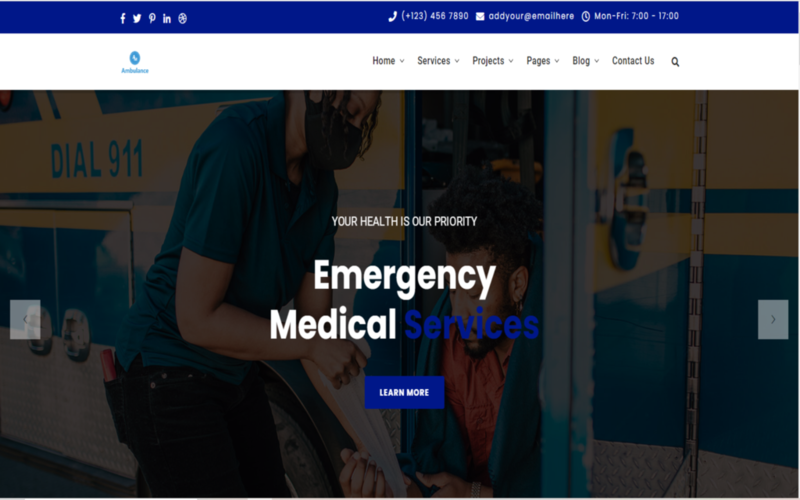This screenshot depicts a slightly distorted webpage, likely due to stretching. The header prominently declares, "Your Health is Our Priority," framing the site’s commitment to medical care. The main hero image on this homepage features a title that reads, "Emergency Medical Services," with 'Services' rendered in a hard-to-read blue font. Below this title, there is a "Learn More" button against a blue backdrop.

In the background, there seems to be an Emergency Medical Services (EMS) scene with some visible details: a vehicle marked with '911,' an EMS paramedic or related personnel, and two individuals—one holding what appears to be a piece of paper, and the other seated.

The top bar of the page includes social media icons, a phone number displayed as "1-2-3-4-5-6-7-8-9-0," a placeholder email "your at email here," and business hours listed as "Monday to Friday, 7-1700 hours." There is a logo, possibly reading "Ambulance," although it’s not very legible.

The site’s navigation menu, placed on a white background with dark blue text, includes links to sections labeled Home, Services, Project, Pages, Blog, Contact, along with a search icon for easy access.